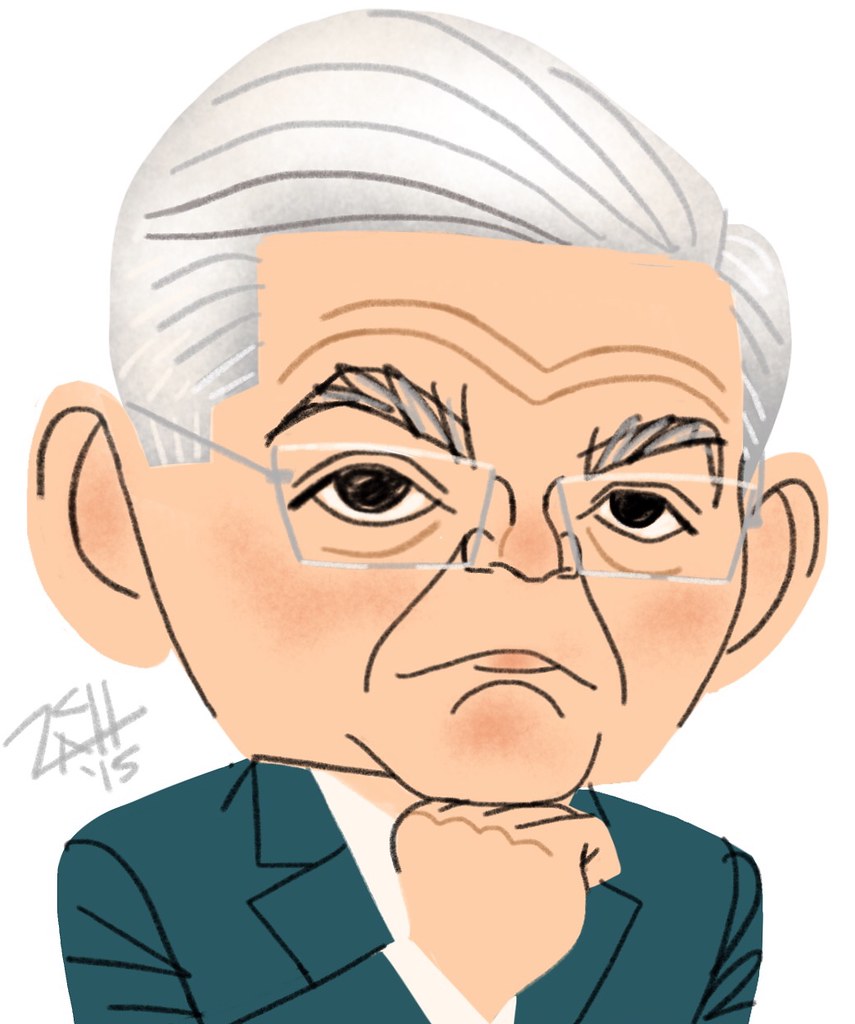The image is a political cartoon featuring Senator Robert Mendez depicted in a whimsical chibi style. Senator Mendez is drawn with an oversized head, nearly as large as or larger than his body. His facial expression is accentuated by rosy cheeks and a rosy chin, along with thin, silver-framed rectangular glasses. His hair is a mix of white and gray, styled in a comb-over, and he has prominent, bushy eyebrows that are gray with black lines. His large ears stick out from his head, and wrinkles on his forehead form into two curved lines, resembling a flattened "M". 

Senator Mendez is portrayed wearing a greenish suit jacket with a white shirt underneath. His right hand is propped up under his chin, with his head resting on it. The background of the drawing is simple and plain white, with no added elements except for an artist's signature over his left shoulder, which reads "ZATS 15" in stylized gray lettering. The overall effect is both endearing and humorous, highlighting the senator's distinctive features.